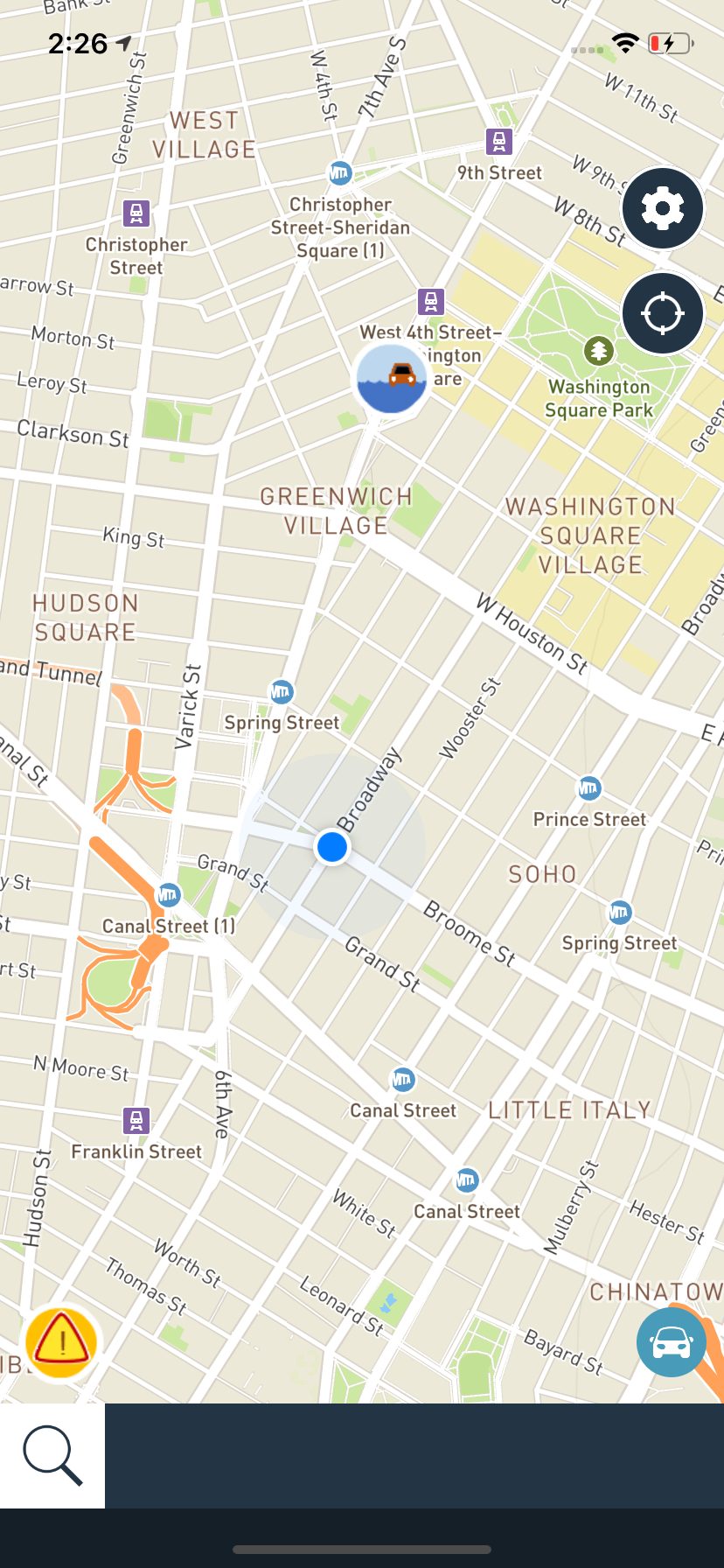A detailed map screenshot from a navigation or ride-sharing app showcases a section of Manhattan, New York City. The time displayed at the top left is 2:26. The top right corner contains signal strength and battery level indicators, showing the battery nearly full and charging. The map vividly portrays streets and neighborhoods, highlighting notable locations such as Greenwich Village, West Village, SoHo, Hudson Square, Little Italy, and Chinatown.

Key landmarks include Washington Square Park, located in the upper-right portion of the map. Several subway stations are marked with the MTA symbol, including Christopher Street, Spring Street, Canal Street, Broadway, and West Houston Street. A blue dot in the center of the map reveals the user's current location, while a larger icon featuring an orange car on a blue background, situated in the lower right, likely signifies a destination or ride-share vehicle.

On the right side of the screen, two circular buttons are visible: a settings icon (depicted as a gear) and a current location symbol (represented as a crosshair). The bottom left corner contains a magnifying glass icon, indicating a search function, and a yellow triangle with an exclamation mark, possibly signaling an alert or warning.

This screenshot provides a comprehensive view of the user’s surroundings in Manhattan, making navigation easier with clearly marked locations and convenient app functionalities.